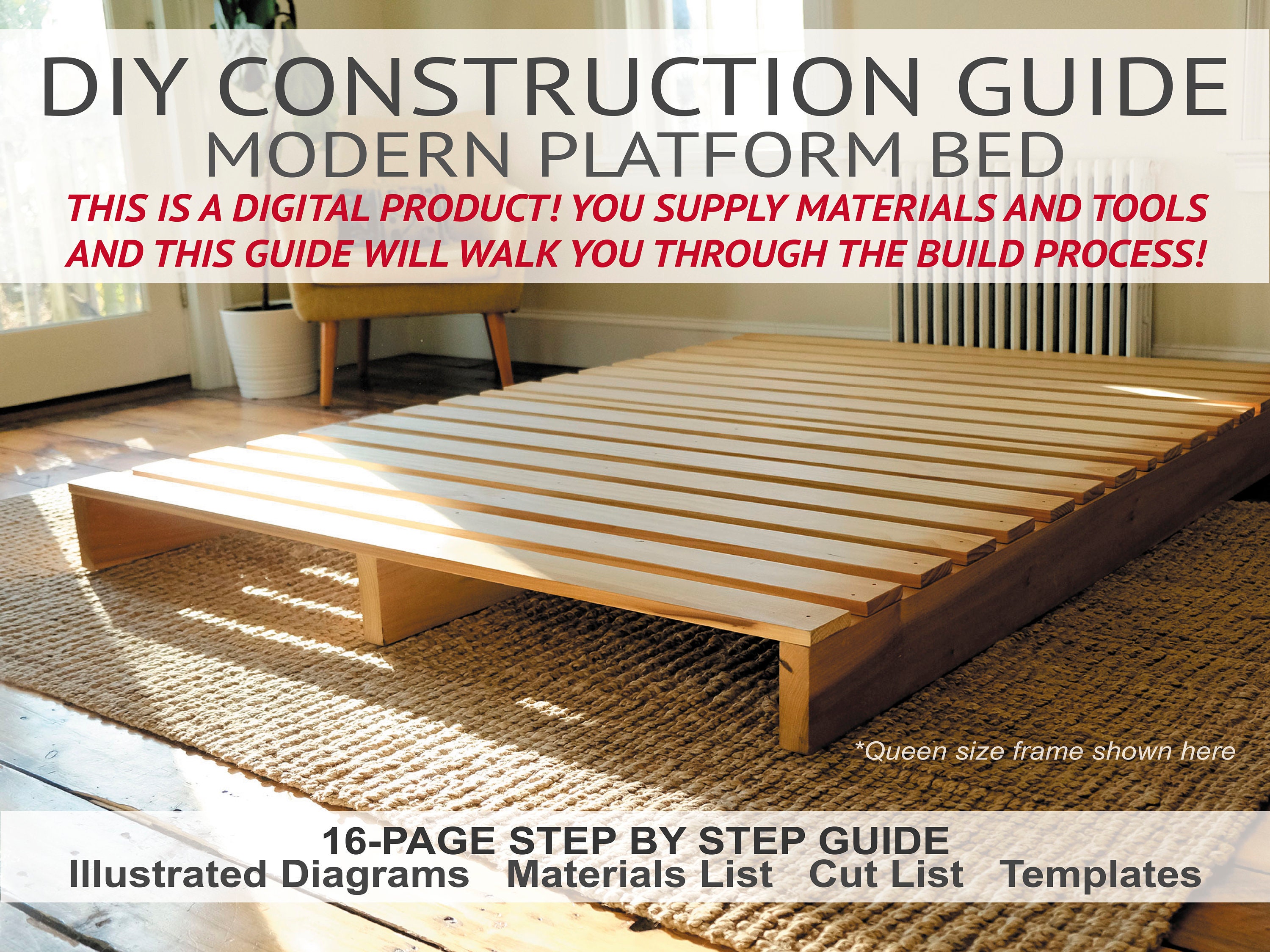This image is a detailed cover of a DIY instruction manual for building a queen-size modern platform bed. At the top, a banner in dark gray font reads "DOI Construction Guide: Modern Platform Bed." Below the banner, in bold red text, it states, "This is a digital product. You supply materials and tools, and this guide will walk you through the build process." The guide is presented as a 16-page step-by-step manual featuring illustrated diagrams, a comprehensive materials list, a cut list, and templates.

An image of the queen-size bed frame, constructed from sheets of timber, occupies the center of the guide. It provides a clear visual reference with the caption, "Queen Size Frame shown here," highlighting the bed's dimensions and design. The bed frame is shown on a sisal or similar natural fiber rug, placed on a medium-tone rustic wood floor. The setting includes aesthetic elements like a tall plant in a white pot, a mid-century chair, painted radiators, and two windows, adding airiness and light to the scene.

The image gives potential builders a preview of the end product while reiterating that they must source their own materials and tools to follow this digital guide and build the bed frame from scratch.